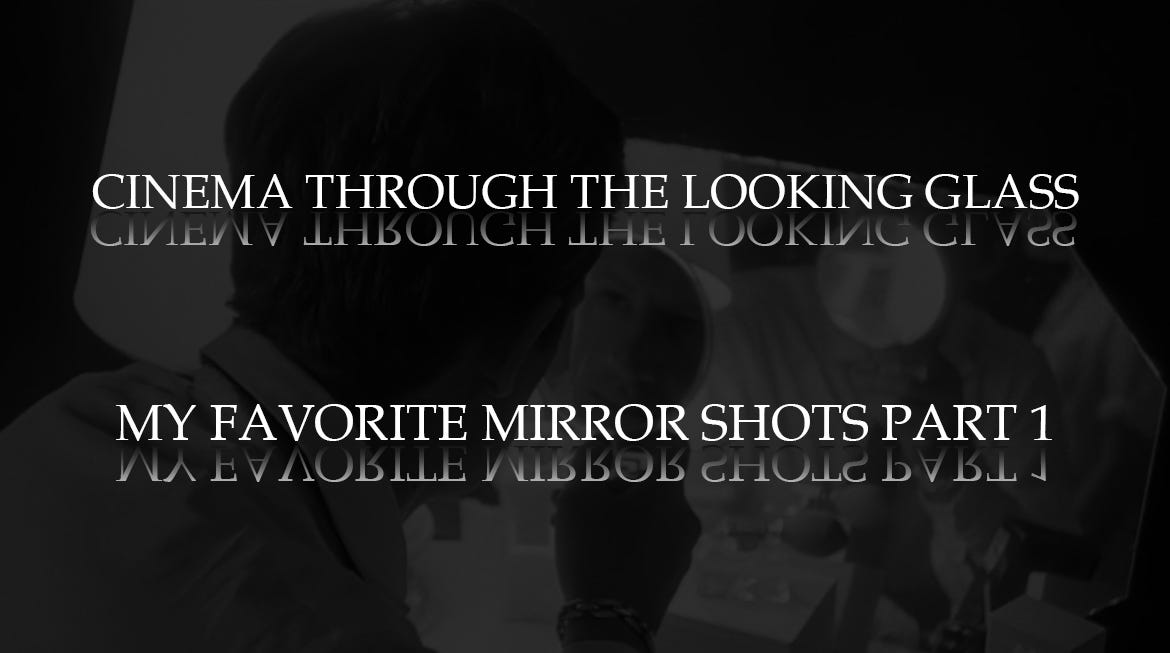The image appears to be a black-and-white screenshot or thumbnail from a YouTube video, likely a video essay about mirror shots in cinema. The background features a dark silhouette of a man standing in profile. He's partially visible, wearing a light-colored collared shirt, with his face and the white collar distinctly standing out. He is also holding a handheld round mirror in which his face can be seen in reflection. Surrounding him are black and white objects that contribute to the overall dark tone of the image.

At the top of the image, in uppercase white letters, it says "CINEMA THROUGH THE LOOKING GLASS," with an upside-down mirror reflection of the text directly below it in a slightly grayed-out color. Similarly, near the bottom of the image, it reads "MY FAVORITE MIRROR SHOTS PART ONE," also with its mirrored reflection underneath. This stylistic choice emphasizes the theme of mirrors and reflections discussed in the video.